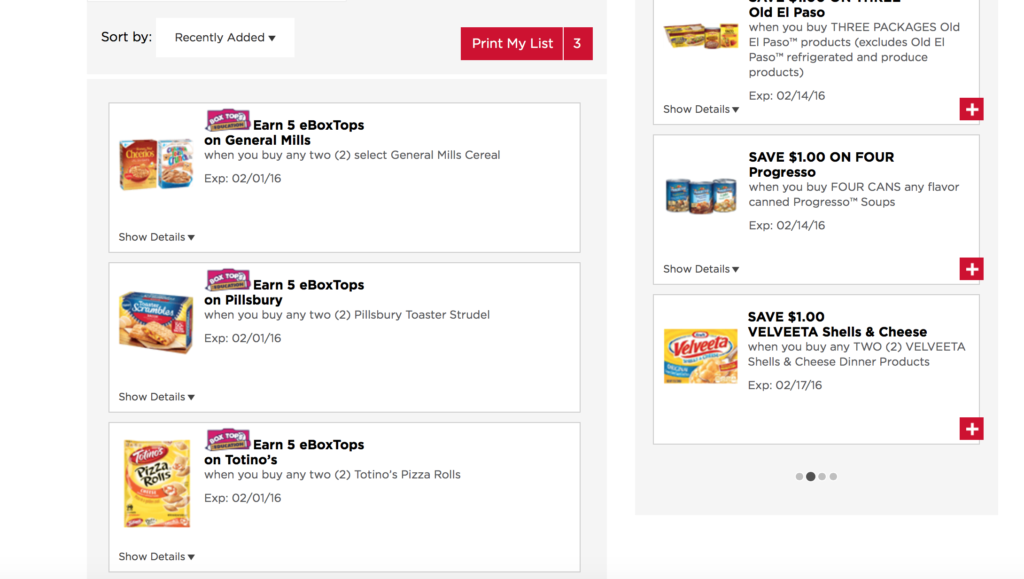The image depicts a digitally organized grocery list interface with various promotional offers from different brands. The screen is divided into two main sections: a left and a right area. 

The left area, shaded in gray, has a dropdown menu at the top left labeled "Sort by," currently displaying "Recently Added." 

On the right side, a prominent red button labeled "Print My List" is visible, accompanied by the number three in parentheses, possibly indicating the number of items selected for the list.

Below, the interface showcases several promotional offers. 

- The first offer highlights General Mills cereals. It features images of a Cheerios box and a Cinnamon Toast Crunch box, with a promotion to "Earn 5 e-box tops" when purchasing any two selected General Mills cereals. The offer is set to expire on February 1, 2016. A "Show Details" button is present underneath this offer.
  
- The second offer is from Pillsbury, promoting an "Earn 5 e-box tops" deal when purchasing any two Pillsbury Toaster Strudels. This section also features an image of Toaster Strudel boxes and an identical expiration date and "Show Details” button as the previous offer.
  
- The third offer is for Totino's products, specifically pizza rolls, under the same promotion terms as the Pillsbury offer.

The right section lists additional promotions:
 
- The first involves Old El Paso products, offering a deal when buying three packages, with an expiration date of February 14, 2016.
  
- The second is a coupon for Progresso soups, offering $1 off when purchasing four cans of Progresso.
  
- The third promotion provides a $1 discount on Velveeta Shells and Cheese, applicable when buying any two Velveeta Shells and Cheese dinner products.

In all sections, the promotional products are visually represented by their respective product packaging images.